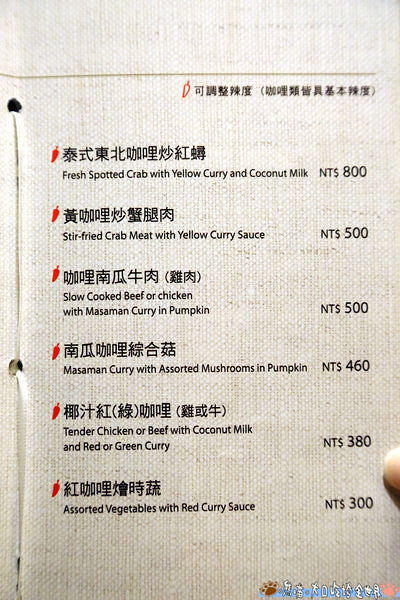The image depicts a laminated menu page with hole punches along one side, suggesting it has been taken out of a binder. The menu is bilingual, featuring six dishes listed in both Asian characters (likely Japanese or Chinese) and English. Each dish is accompanied by its price in New Taiwan Dollars (NT$). The first item is "Fresh Spotted Crab with Yellow Curry and Coconut Milk," priced at NT$800. This is followed by "Stir-fried Crab Meat with Yellow Curry Sauce" for NT$500. Next, the menu offers "Slow-cooked Beef or Chicken with Massaman Curry and Pumpkin" also at NT$500. The fourth dish, "Massaman Curry with Assorted Mushrooms and Pumpkin," is priced at NT$460. "Tender Chicken or Beef with Coconut Milk and Red or Green Curry" follows, costing NT$380. The final item is "Assorted Vegetables with Red Curry Sauce" for NT$300. Additionally, each dish is marked with a spicy pepper icon to the left, and a finger is visible in the image, indicating someone is holding the menu page.